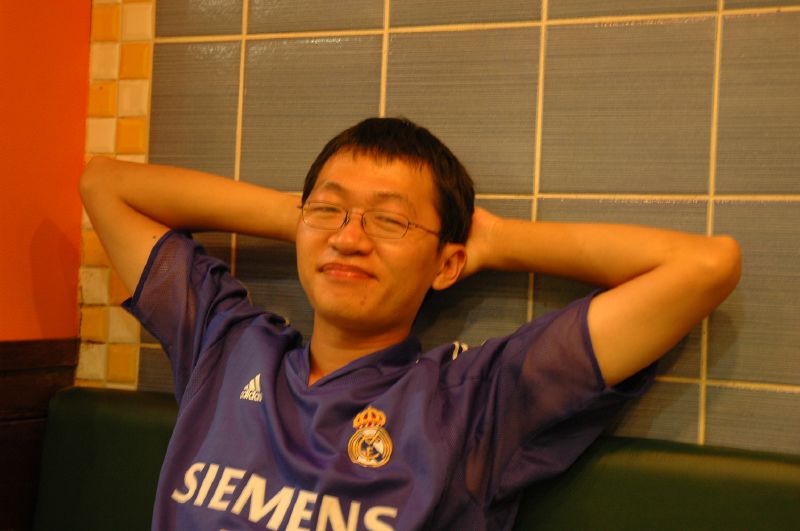The color photograph features an Asian man with short black hair and glasses, sitting relaxed in what appears to be a restaurant booth. His hands are positioned behind his head as he leans back against a green upholstered seat. He is wearing a purple, short-sleeve soccer jersey adorned with a white Adidas logo on the upper left side, a golden circular club emblem with a crown on the right, and "Siemens" spelled out across the front. The man, who has a slender build, is giving a contented, close-lipped smile. The background reveals a gray tiled wall, with sections of smaller white and yellow tiles to the left and an adjacent orange wall, indicating that he is situated in the corner of the room. Overall, he appears relaxed and content, embodying the demeanor of a dedicated soccer fan.